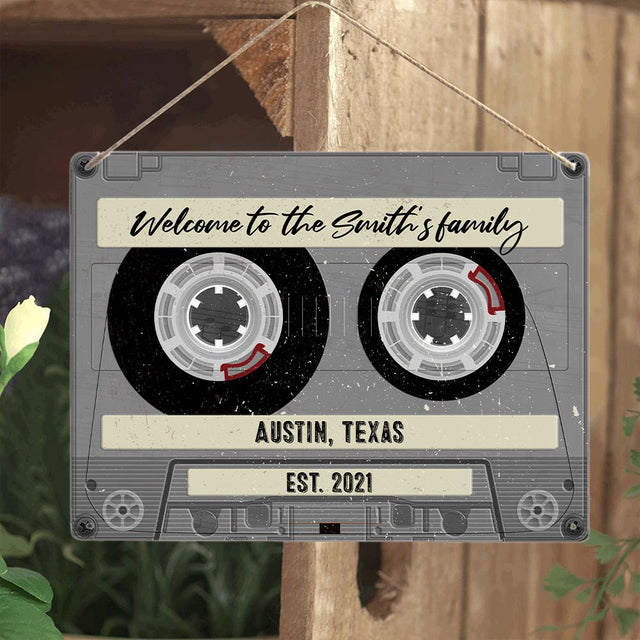The image features a rustic wooden structure, possibly a fence or a box, made of natural, unstained brown wood. Only a portion of the wood is visible. On the left side of the structure, a delicate, light yellow flower resembling a tulip adds a touch of color and nature to the scene.

Hanging from the wooden structure is a gray sign designed to look like an old cassette tape. The top of the sign displays the cursive text "Welcome to the Smiths Family" in elegant black lettering. Just below the reel-to-reel detail of the cassette tape, the words "Austin, Texas" are prominently written in uppercase black letters. Beneath that, the establishment year "Established 2021" is also showcased in bold, uppercase black letters. The combination of the vintage cassette design and the welcoming message creates a charming and nostalgic decoration.